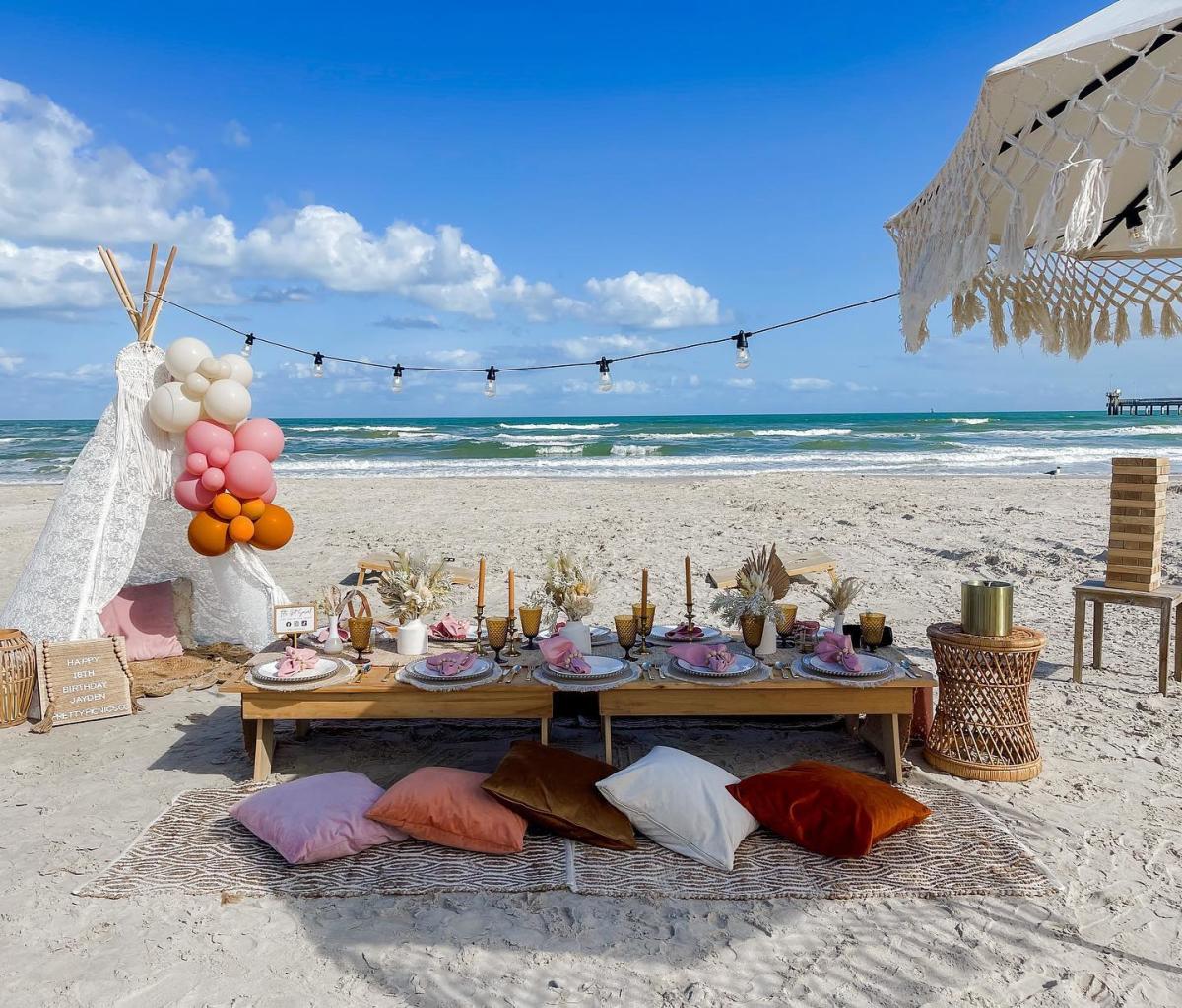The color photograph depicts a vibrant beachfront celebration against a backdrop of a bright blue sky with puffy clouds and an expansive ocean view, with a pier extending into the water on the far right. Central to the image is a low, light brown wooden table set for five, adorned with white plates, silverware, and amber-tinted glasses. The table features tall taper candles and is bordered by an array of pillows in hues of dark red, light brown, peach, and pink, all resting on a light beige rug.

Overhead, a string of lights drapes between structures, providing a festive ambiance. To the left of the table stands a white teepee, decorated with a cluster of white, pink, and orange balloons, alongside a barely visible sign that reads "Happy 18th Birthday, Jaden." A canopy is visible off to the right, where a smaller end table holds a large pillar candle set in a metal container. At the extreme right edge of the image, there is a wooden table holding a Jenga game, ready for entertainment. This picturesque setting, complete with an umbrella providing shade to part of the scene, captures the essence of a joyful beachside gathering.